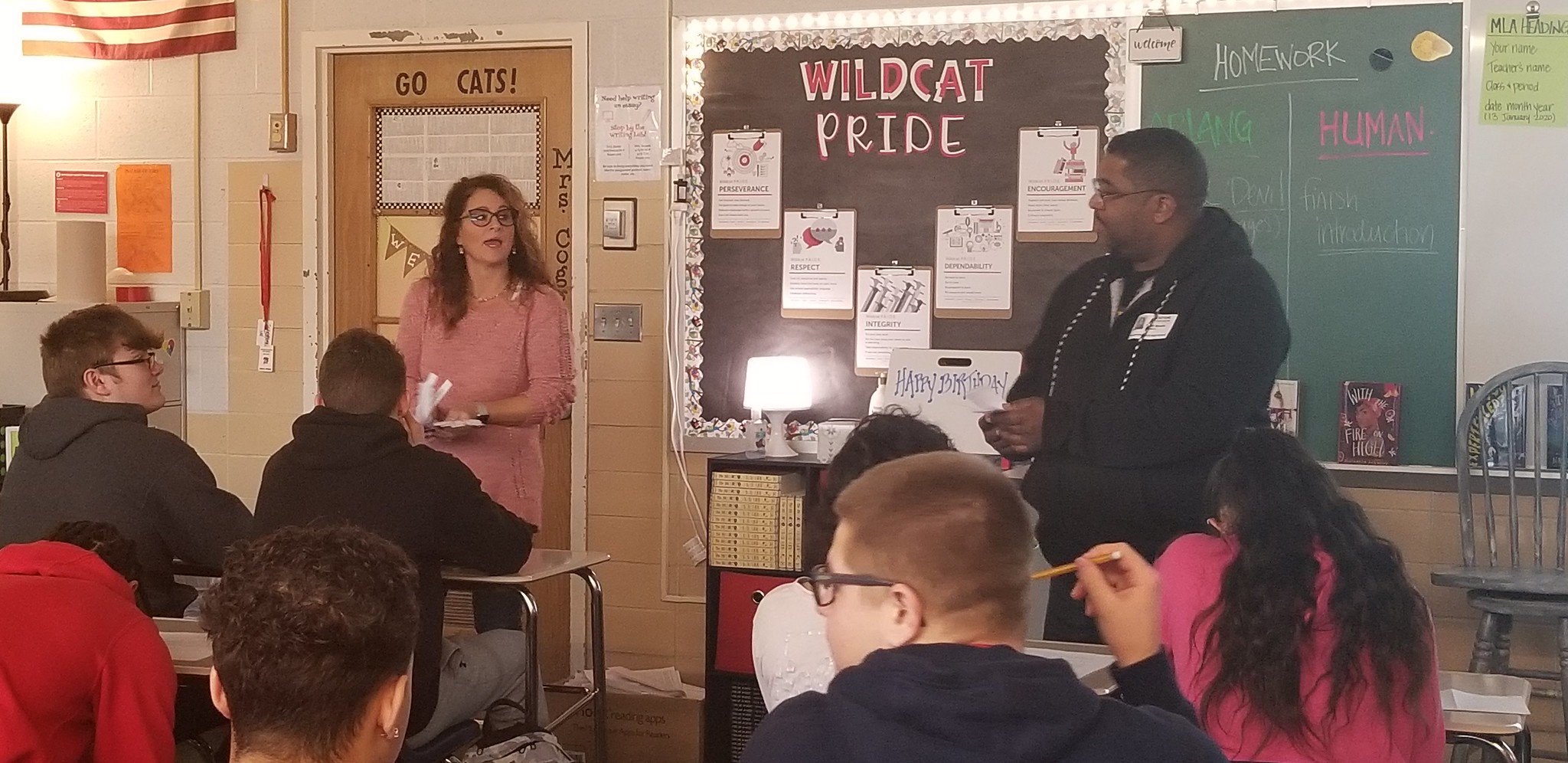In this high school classroom, the photograph captures a detailed scene with various elements. The hardwood flooring sets a warm tone beneath the students' desks, where teenagers focus intently on the front of the room. At the bottom of the image, we see the backs of several students’ heads. Dominating the center is a black man dressed in a black hoodie with black and white striped pull strings, suggesting his role as a guest speaker or presenter. His visitor pass or name tag is visible on his chest. To his left, near the door, stands a white woman wearing a pink top and glasses, with light brown frizzy hair. She appears to be speaking to him. 

Behind them, the chalkboard and whiteboard are covered with messages like "Go Cats!" and "Wildcat Pride," likely school mottos. Additional details include the colors red, black, gray, brown, pink, and green scattered throughout the room, adding vibrancy to the setting. The scene, set in the middle of the day, is alive with educational and collaborative energy.